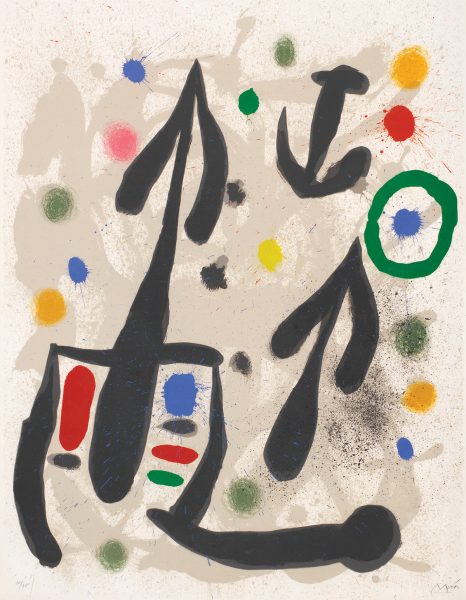The abstract painting, set against a beige background, features a dynamic composition of arrows and bold black strokes reminiscent of Asian calligraphy. There are three prominent arrows: the largest one points up on the left, another points up towards the sky, and a smaller one points downward. The most substantial arrow is bordered by a black line that culminates in a ball on the right side, accompanied by diverse splashes of color such as reds, blues, blacks, and greens. Among the intricate details, one arrow resembles an exclamation point with a black dot beneath it, while another smaller arrow at the top bears a striking resemblance to a boat anchor. Surrounding these arrows are various colorful paint splatters and swoops in shades of green, yellow, pink, and orange, with some forming circular patterns. Scattered brown specks add to the chaotic beauty of the scene. The painting, evocative of Kandinsky’s style, concludes with a partially legible signature starting with 'M' in the bottom right corner.